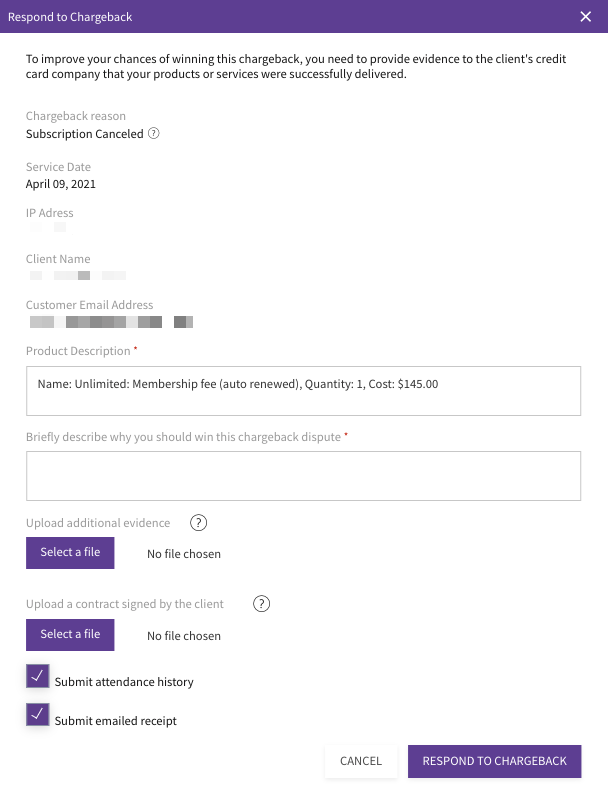The image is a vertically oriented screenshot of a webpage, likely taken on a tablet. At the top of the page, there's a prominent purple banner with white text that reads "Respond to Charge Back." The background of the page is predominantly white, and the select buttons are distinguished by their purple color with white text.

Below the banner, instructions are provided: "To improve your chances of winning this charge back, you need to provide evidence to the client's credit card company that your products or services were successfully delivered." The charge back reason listed is "Subscription cancelled," with the service date noted as April 9, 2021.

Further down, there are fields for the IP address, client name, and customer email address, all of which are pixelated to protect the customer’s privacy.

In the product description section, details read: 
- Name: Unlimited Membership
- Fee: Auto Renewed 
- Quantity: 1 
- Cost: $145 

Below these details, there's an empty text box accompanied by the prompt: "Briefly describe why you should win this charge back dispute." Additionally, there's a section for uploading additional evidence, featuring a file upload box that currently states "No file chosen."

Another area prompts the user to "Upload a contract signed by the client," with a file selection box present, but also stating "No file chosen."

Towards the bottom, there are two checkboxes with purple check marks, labeled "Submit Attendance History" and "Submit Emailed Receipt." Finally, at the lower right corner of the page, there are two buttons: a "Cancel" button and a "Respond to Charge Back" button.